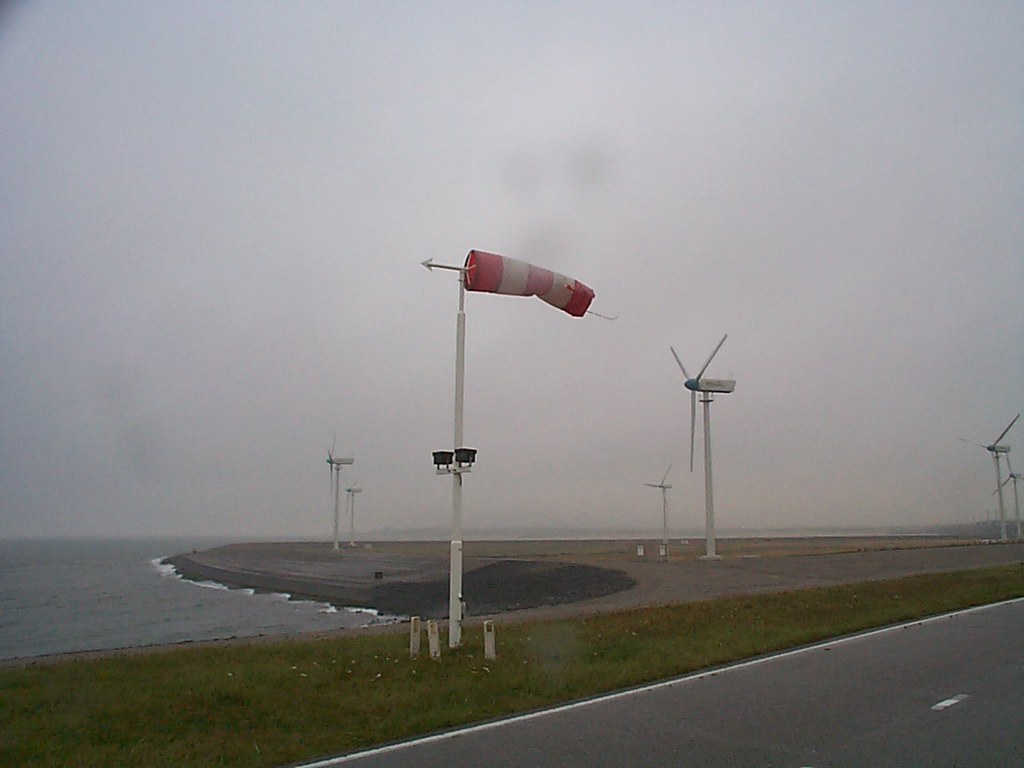This outdoor photograph captures a cloudy day at a wind farm located near a shoreline, possibly overlooking an ocean, sea, or lake. Central to the image are six large wind turbines standing tall in a vast, dirt-covered area. In the foreground, spanning from the lower right, runs a gray asphalt road bordered by patches of green grass dotted with dandelions. Adding detail, a series of short poles extend from the ground, accompanied by a taller pole that supports a red and white windsock, which also serves as a weather vane. Additionally, there are two lamps positioned beneath the windsock, likely used to illuminate it during nighttime or inclement conditions. Prominently featured colors in the image include gray, pink, red, white, black, and green, which collectively enhance the atmospheric, overcast setting.